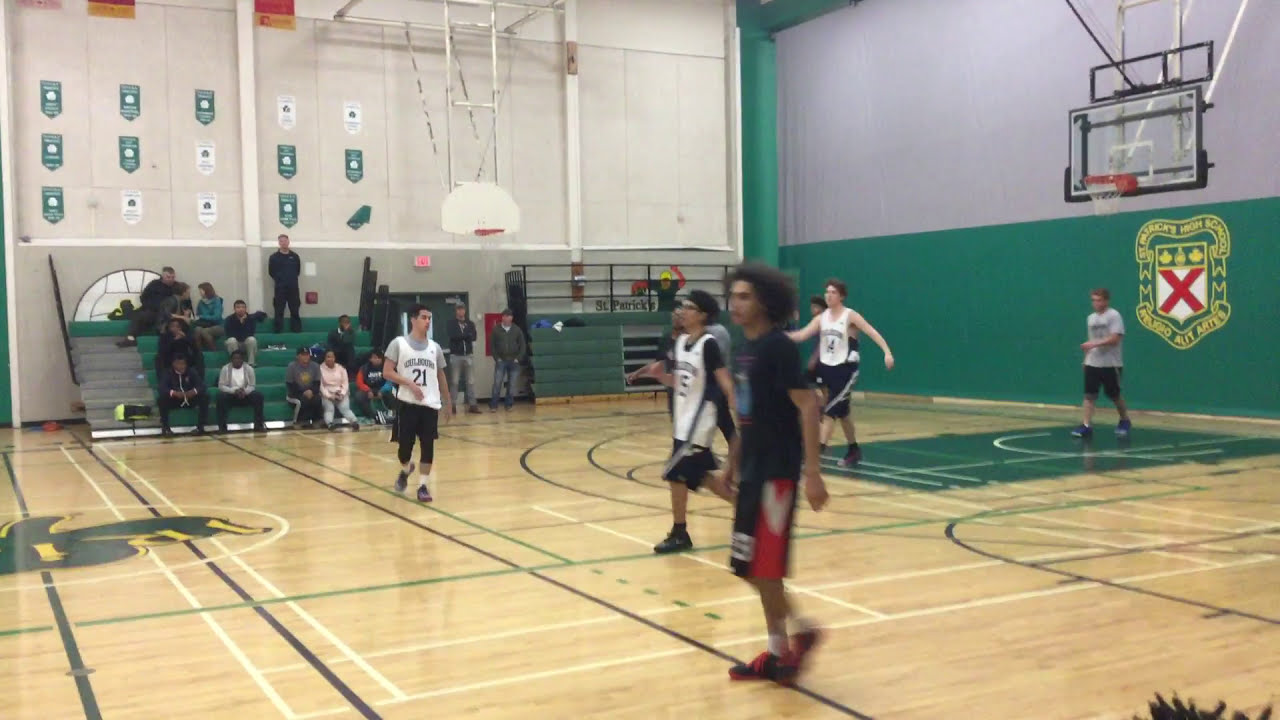This horizontally aligned rectangular photograph captures an indoor basketball game in a gymnasium with high ceilings and primarily white walls. The lower half of the wall on the right is green, featuring a badge with an X in the middle, while the upper part is gray. The gym floor is light brown with an assortment of stripes in dark blue, green, yellow, and white.

In the center foreground, there is a blurry image of a young man wearing a dark short-sleeved shirt and black, red, and white shorts, his short black hair evident despite the blur. On the court surrounding him, there are approximately five to six players, most of whom are dressed in white jerseys with black shorts and lettering, though the text on the jerseys is difficult to discern. 

The upper right corner of the image shows a basketball hoop attached to a glass backboard. To the left, there are green and gray bleachers with about ten spectators, one of whom is standing on the top row. Behind the bleachers are alternating green and white banners hung on a white wall. The overall scene is dynamic, suggesting motion, as several figures appear blurry, indicating the fast-paced action of the game.